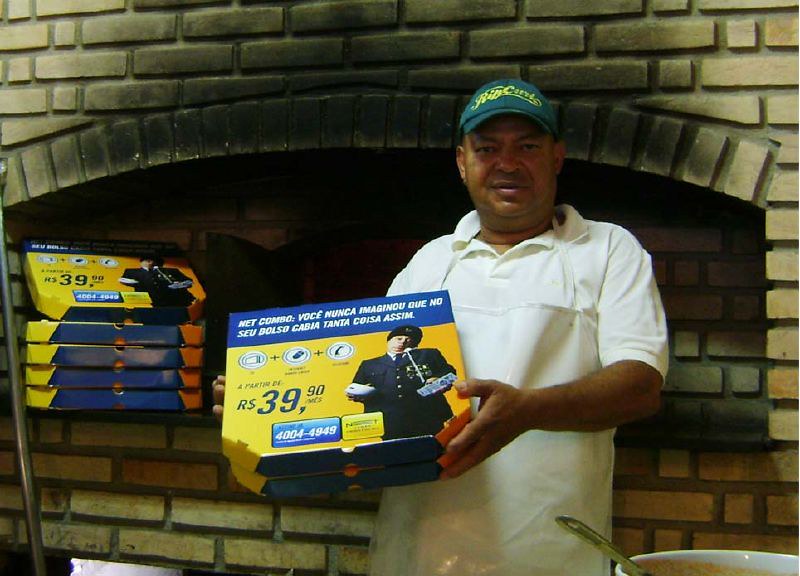In this photograph, a man, who appears to be of Latin or Mediterranean descent, stands in front of a large, tan brick wood-fired pizza oven. He is dressed in a white polo shirt, a white apron, and a green cap with yellow lettering in a foreign language. The pizza oven, prominently made of large bricks and featuring smoke stains above its opening, extends from the left to the right side of the picture. The man holds two pizza boxes, which he is displaying to the camera. These boxes are blue and yellow, featuring an advertisement in Spanish that mentions a combo deal priced at 39.90. The boxes also depict a figure in a blue uniform, resembling a policeman, holding a phone. Behind the man is a stack of similar boxes, and to his side, there is a white bucket and a large pizza paddle. In front of him, a white pot with a large spoon, likely containing pizza sauce, completes the scene.